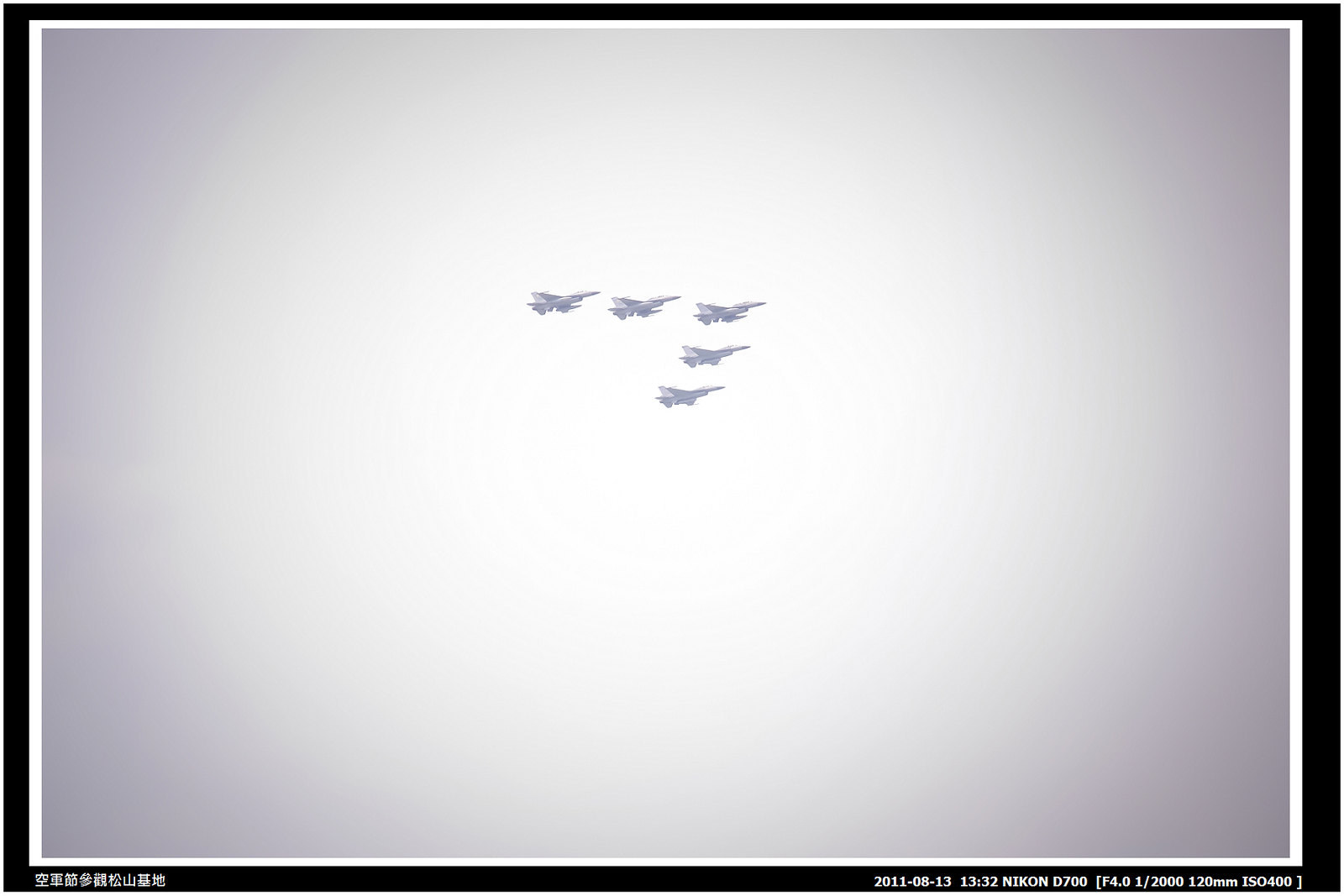This black and white image features five intricately detailed fighter jets flying in a V formation. The aircraft, potentially F-16s, showcase wings, fins, and a pointed nose, consistent with fighter jet designs. The planes are arranged with three on top and two beneath, all pointing eastward, creating a striking triangular pattern in the clear, cloudless sky. The photograph exhibits a gradient, darker gray at the corners, gradually becoming lighter toward the center. Encased in a black outer border and a white inner border, the image contains Chinese or Japanese text in the bottom left corner and a timestamp in the bottom right, reading "2011-08-13, 1300 hours and 32 minutes." Captured with a Nikon D700, its settings included F 4.0, a shutter speed of 1/2,000, 120mm focal length, and ISO 400.